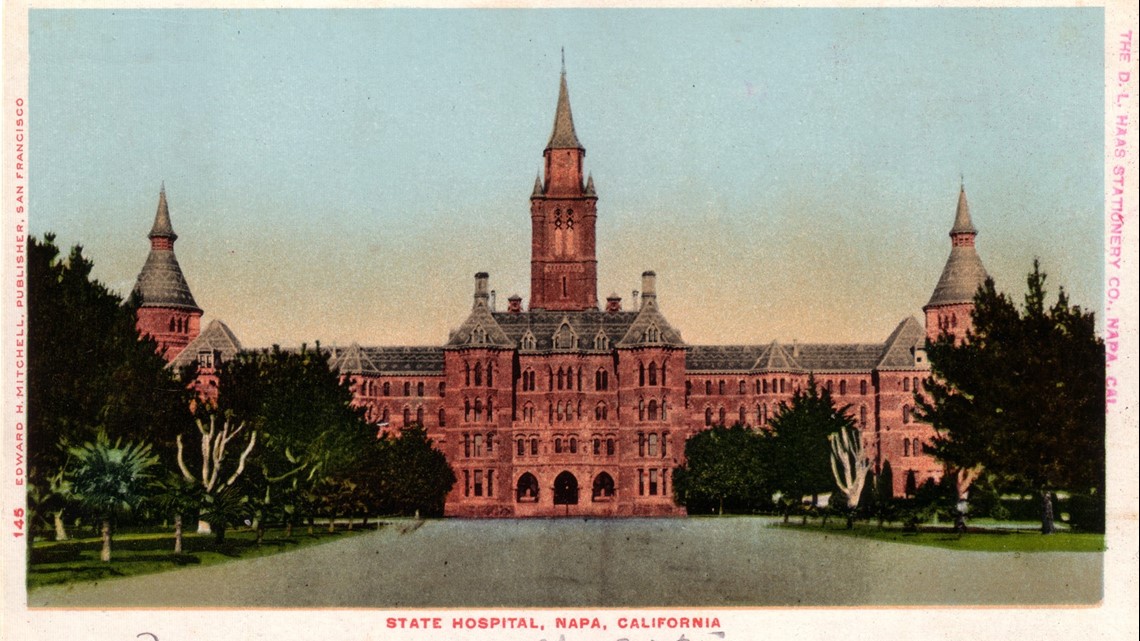This vintage postcard of the State Hospital in Napa, California showcases a large, reddish-brown building that spans nearly the width of the card. The grand, symmetrical structure is accentuated by three prominent towers: one at each side and a taller, central tower. Its architecture, resembling that of a Gothic church or monastery with a quite fancy entrance, stands out. The postcard features a white border with captions identifying the location at the bottom and additional words on the sides. The building is depicted with multiple windows and intricate details, including lines with circular tops, giving it a castle-like appearance. A broad stone sidewalk runs from the foreground towards the building, flanked by lush trees, including distinctive palm trees, which frame the pathway leading up to the impressive State Hospital. The grounds are well-maintained with expansive grass areas under the trees, enhancing the picturesque and historical charm of the scene.